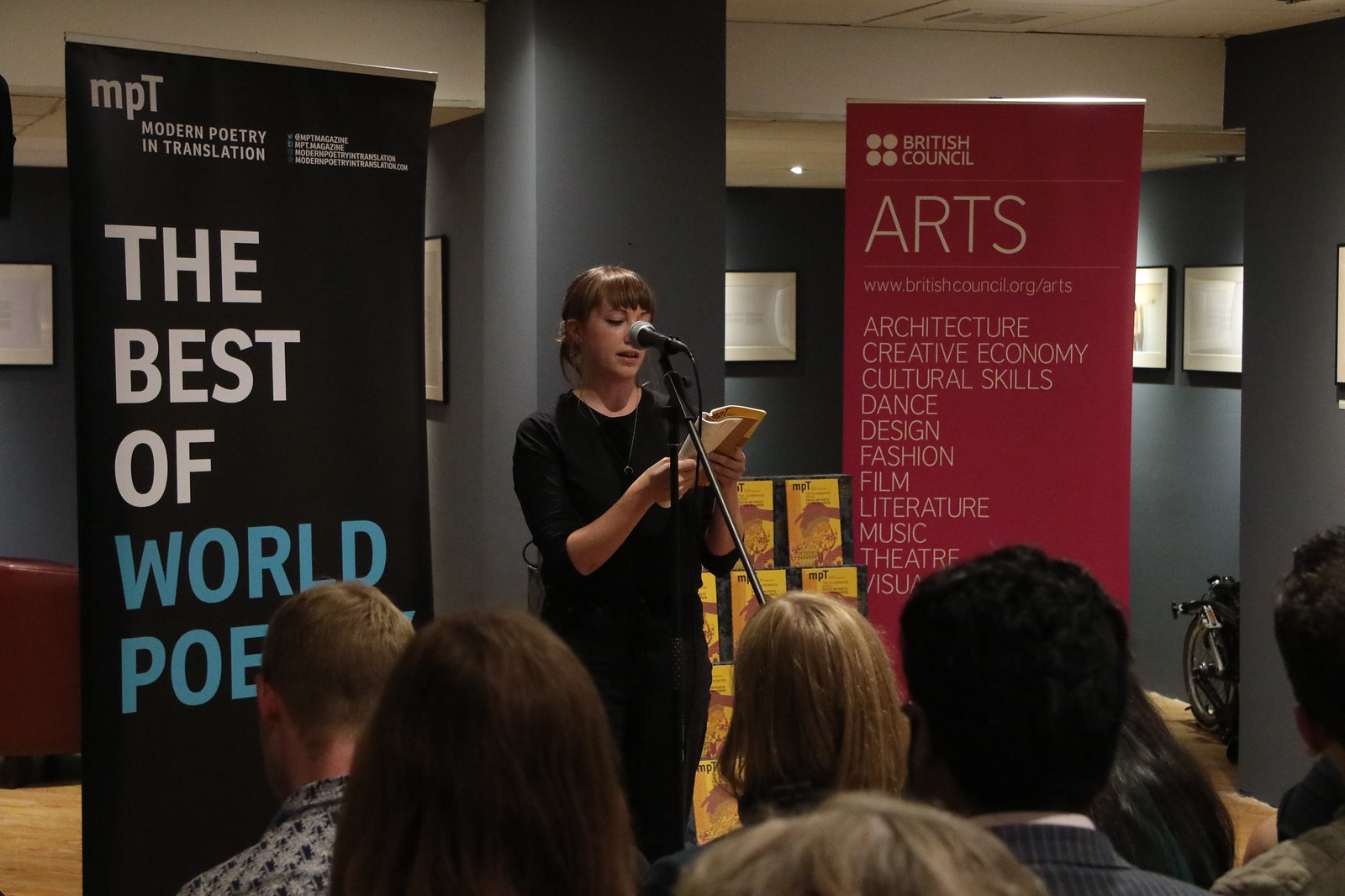In the image, a woman dressed in an all-black outfit and black undershirt stands at a microphone, reading from a yellow book with white pages. She has dark hair and is using a black microphone with a silver mouthpiece, held by a black microphone stand. In the audience below, individuals are seated with varying hair colors: the far left person, wearing a gray shirt with black symbols, has brown hair, followed by another person with brown hair, a person with blonde hair, and then a man in a gray and white pinstripe suit with a white undershirt, who has black hair. More people with dark hair are also visible.

Behind the woman, the walls are gray. To the left, a black sign with white and blue text reads, "MPT, Modern Poetry in Translation, The Best of World Poetry." On the right, a red banner with white text and four white dots states, "British Council Arts, www.britishcouncil.org/arts," followed by a list including architecture, creative economy, cultural skills, dance, design, fashion, film, literature, music, theater, and visual arts. There is a wheelchair in the corner, and the floor appears to be brown wood. Additionally, a shelf in the background holds multiple books, resembling the yellow book from which the woman is reading.